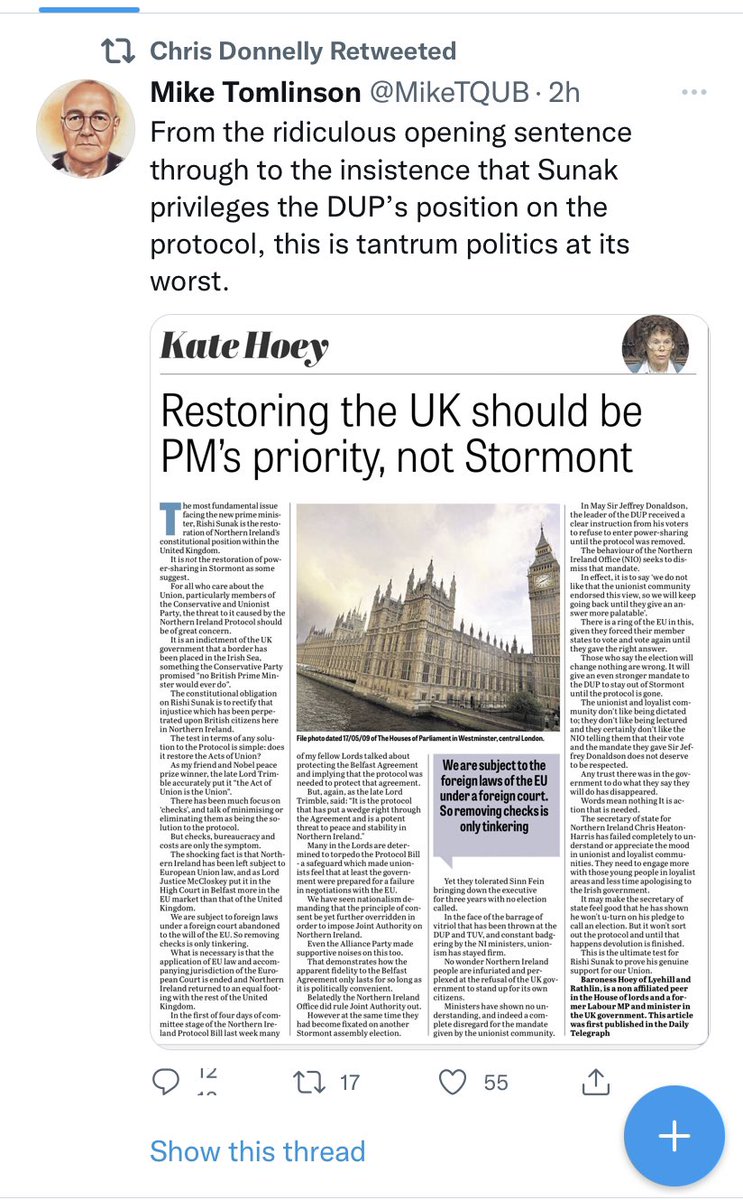On the webpage displayed on a smartphone, the screen captures a retweeted tweet by Chris Donnelly. At the top, beside the retweet icon, is the small avatar of a man wearing glasses and a black shirt or coat. This is Mike Tomlinson, with the handle @MikeTQUB, followed by a timestamp marked as "2H" indicating the tweet was made two hours ago.

The tweet reads: "From the ridiculous opening sentence through to the insistence that SUNAT privileges the DUP's position on the protocol, this is tantrum politics at its worst."

Below the tweet, the rest of the screen is filled with a newspaper article. The article headline reads, "Restoring the UK should not be PM's priority, not Stormont," attributed to Kate Hoey whose avatar, a woman wearing glasses and a white-collared top, is also displayed. The text of the article is organized into four columns with the British Parliament building’s image occupying the top half of the middle two columns.

At the bottom of the page, social media interaction icons are displayed: a speech bubble icon with the number "12" indicating replies, a retweet icon with "17", a heart icon showing "55" likes, and an upload or share icon. To the left, there's a "Show this thread" label in blue, while on the right, a large blue circle with a plus sign is prominent, likely meant for writing a new tweet.